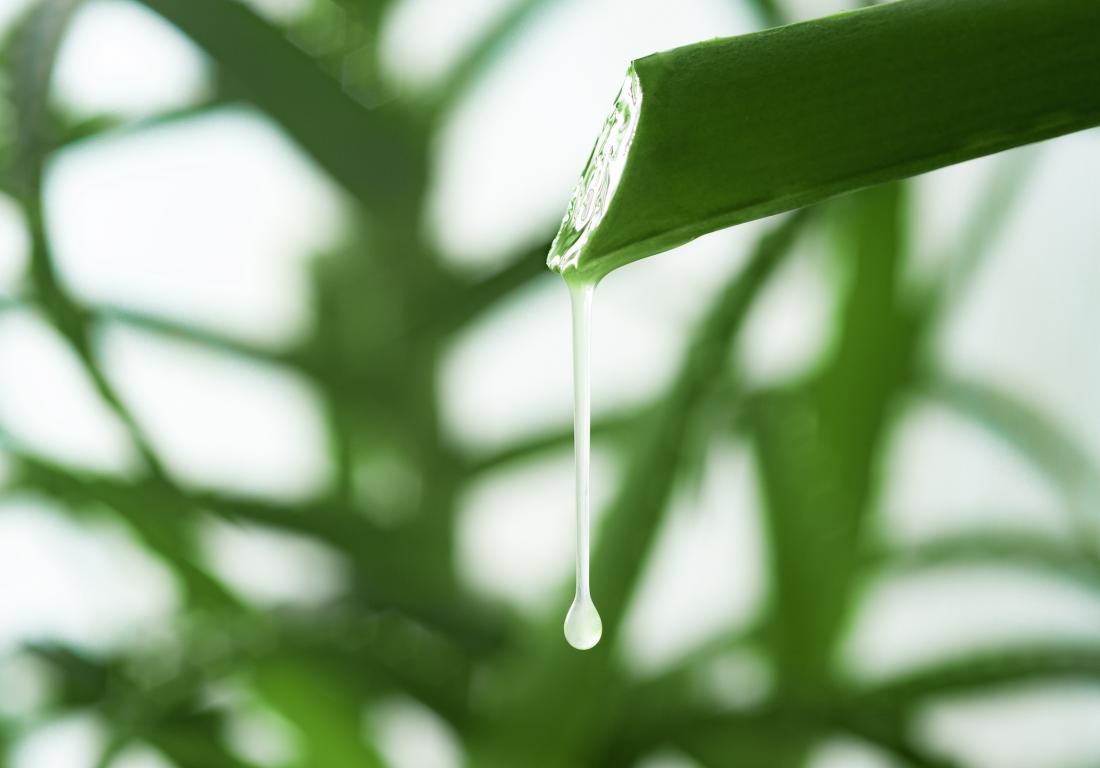The image is a close-up of a bright green aloe plant, prominently featuring a single stalk that extends from the top right corner to the center of the photo. The stalk has been cut at an angle, revealing the plant's inner white tissue and allowing aloe vera juice to drip visibly. The drip forms an inch-long string of liquid ending in a teardrop shape. The background consists of a blurred mix of white and various shades of green, hinting at multiple aloe leaves and stalks. This blurriness ensures the focus remains entirely on the cut aloe stalk and the dripping juice in the foreground.